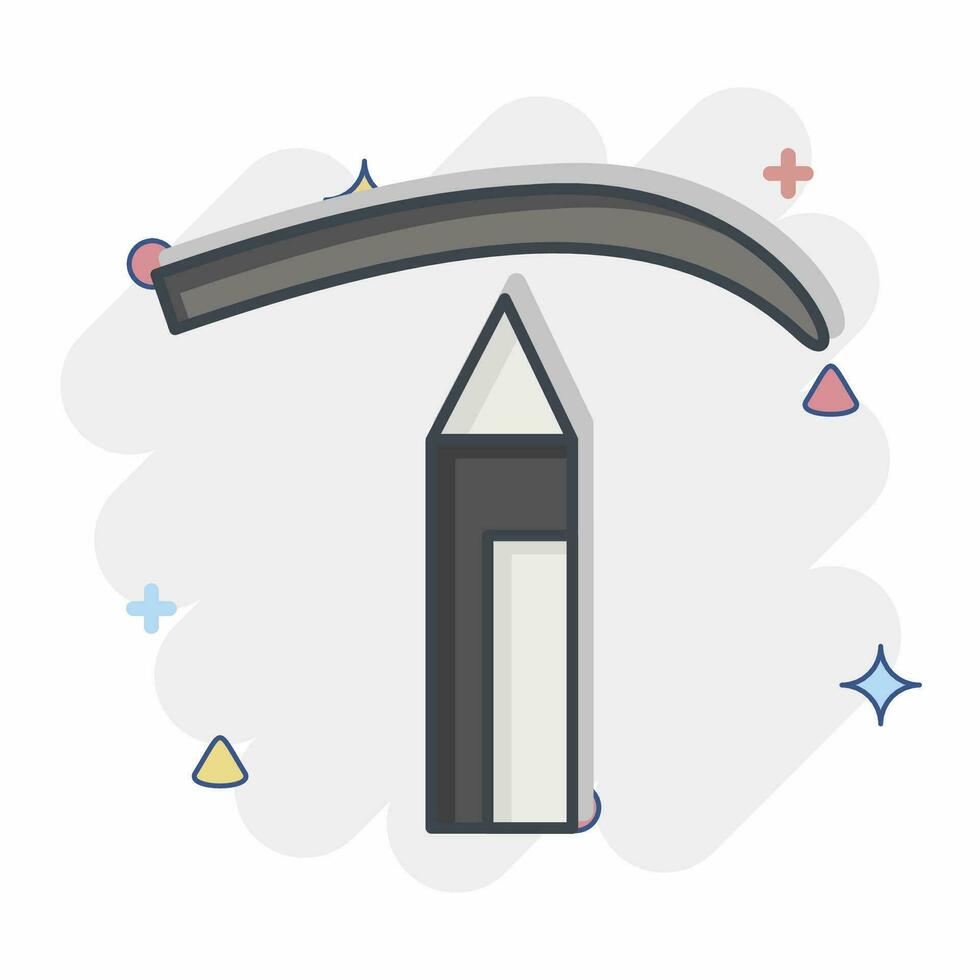This image appears to be a digital illustration or a cartoon with a simplistic, stylized design. Dominating the center is a vertically-oriented, house-shaped figure that bears resemblance to both a pencil and a building. The structure features a black outline with a gradient of dark gray to light gray, culminating in a white tip. At its top, there is a white triangle that mimics a roof. There is also an overhead, curved shape resembling an eyebrow or a banana in dark gray.

The background is minimalistic, comprising a light gray smear or splotch, giving a painted effect. Scattered around the central figure are various small, colorful icons: a yellow triangle, a pink rounded triangle, a pink circle, an orange plus sign, a blue plus sign, and a blue star. These icons are outlined in different colors, adding a whimsical touch to the scene.